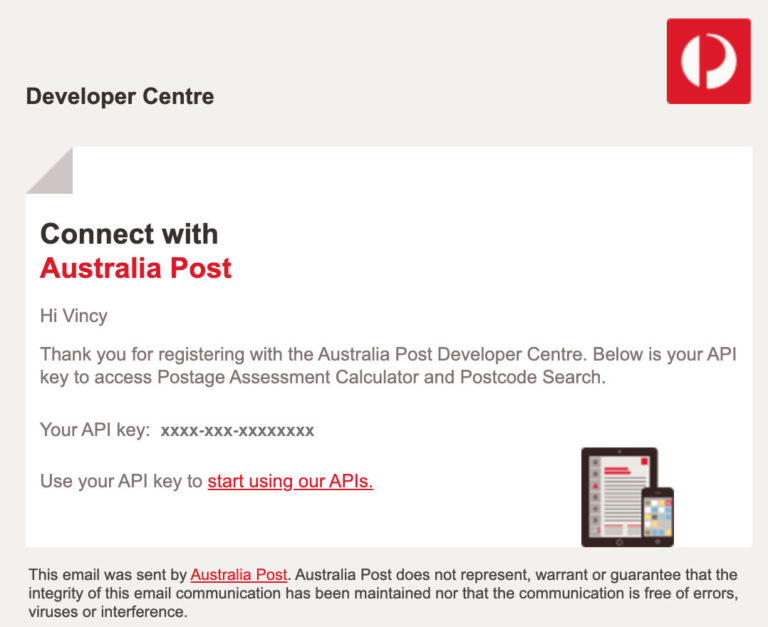The image features a gray square with a white box inside it. In the upper left corner of the gray square, the text "Developer Centre" is displayed. On the opposite corner, there's a red box with a white "P" encircled. Inside the white box, the upper left corner has a bent-over section, resembling a folded paper triangle.

The first text inside the white box reads "Connect with" in black, followed by "Australia Post" in red on a new line. Below, a message says, "Hi Vincy, thank you for registering with the Australia Post Developer Centre. Below is your API key to access postage assessment calculator and postcode search." The API key is represented as "XXX-XXX-XXXX-XXXX." Another note reads, "Use your API key 2," in black text. There’s a red hyperlink saying, "start using our APIs."

Further down, it states, "This email was sent by Australia Post," in red with a hyperlink. The final segment in black text clarifies that "Australia Post does not represent, warrant, or guarantee that the integrity of this email communication has been maintained, nor that the communication is free of errors, viruses, or interference."

Additionally, within the white box, there is an image of a tablet computer with a vertically positioned cellphone in front of it.